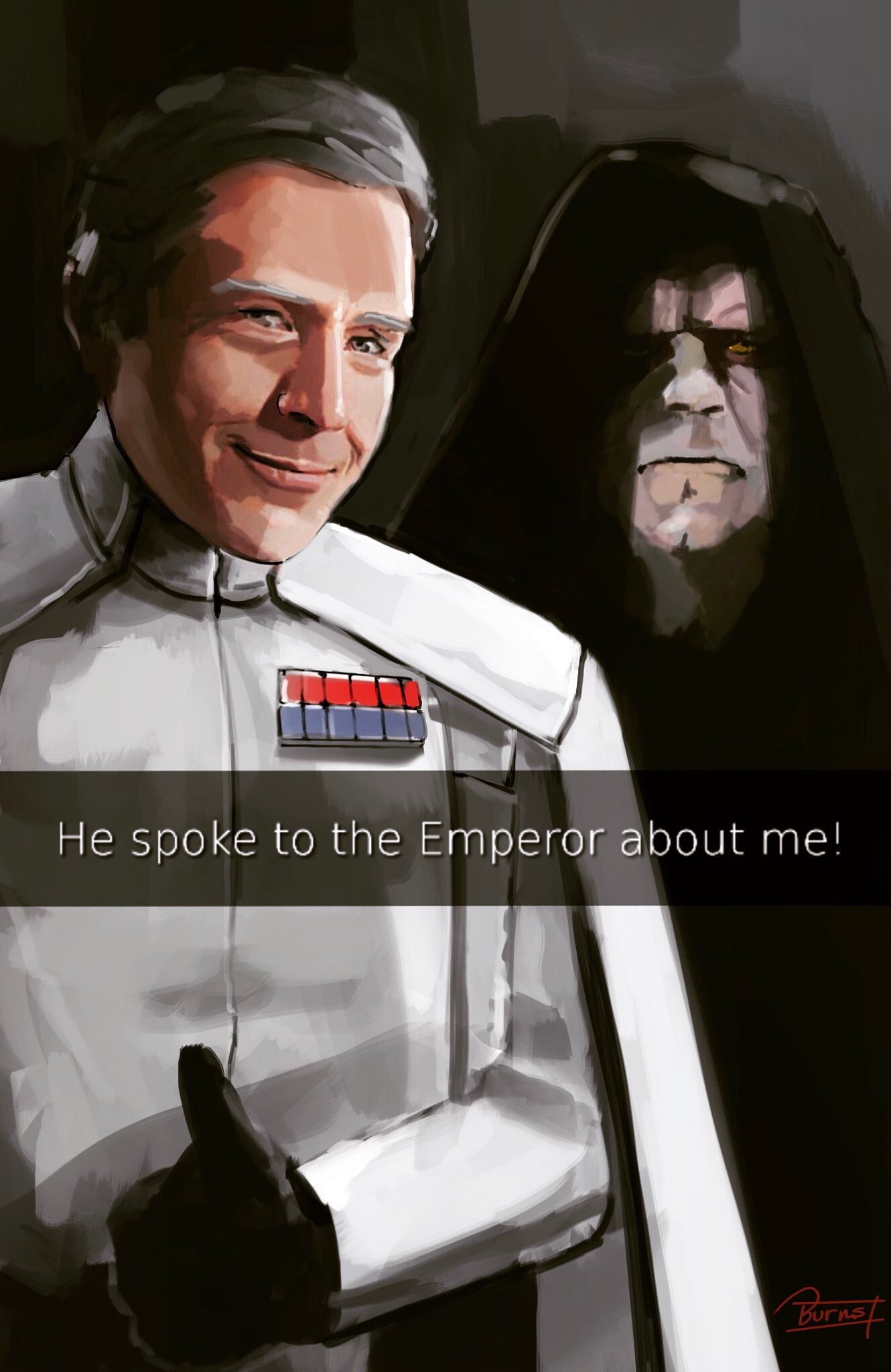The animated image depicts two characters taking up the majority of a vertical rectangle. On the left is an older man with short grayish-brown hair and gray eyebrows, smiling slightly. He is dressed in a white uniform resembling a general's attire, complete with a flowing white cape and black gloves. Prominently displayed on his left chest is a rectangular badge, the top half of which is red and the bottom half gray with vertical grid marks. The man is giving a thumbs-up with his left hand, which is gloved in black. 

To the right stands Emperor Palpatine, recognizable from the Star Wars franchise, though partially obscured. His face is white and he wears a black hood, with his body blending into the dark background. The image bears a watercolor painting style, adding an artistic touch.

Across the middle of the image stretches a black strip with white text that reads, "He spoke to the Emperor about me!" Above the heads of the characters, the background fades from gray on the right to black on the left. Additionally, at the bottom of the image, there is a faint signature, possibly reading "Ciberno," indicating the artist.